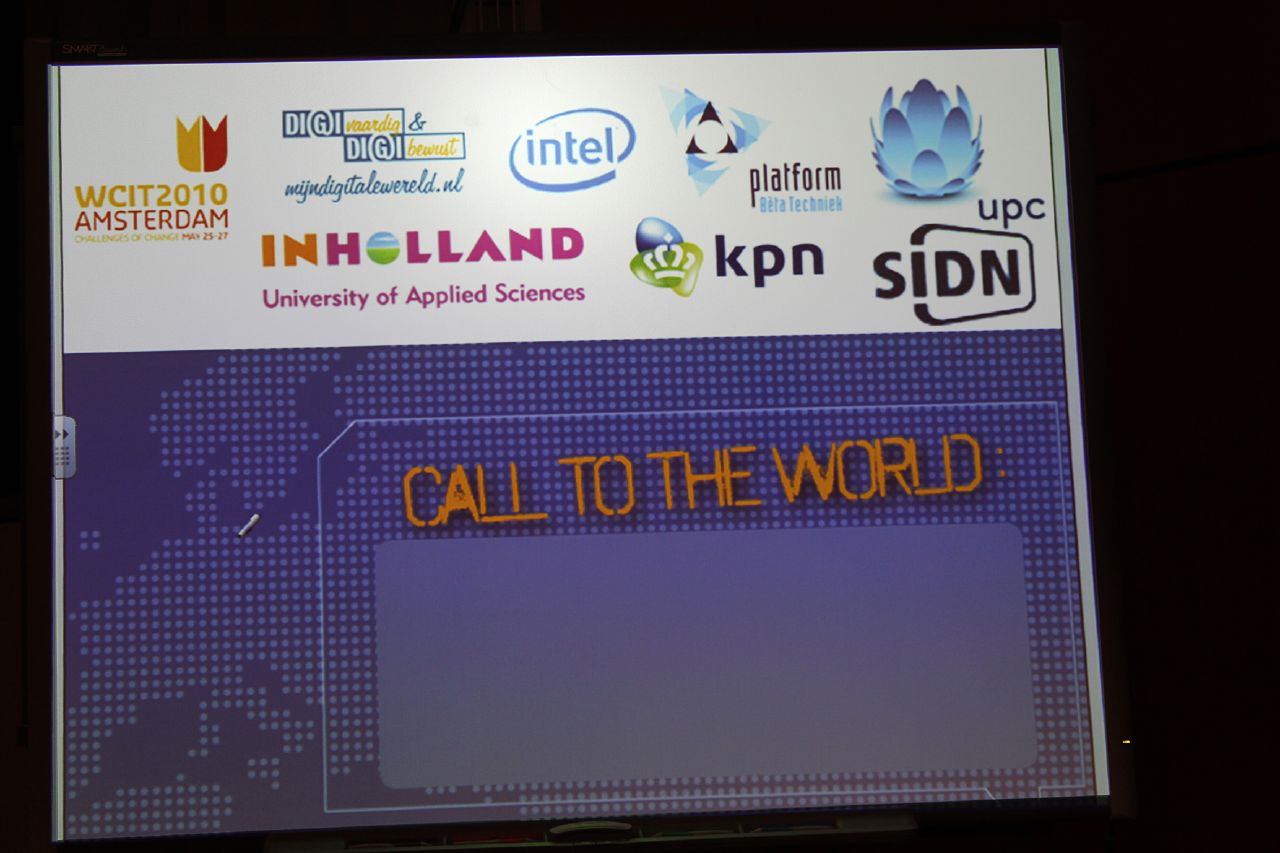The image depicts a projection screen in a dark room, where the backdrop is entirely black, possibly indicating a presentation setup. The screen is notably divided into two distinct sections. The upper portion, smaller than the lower, features a white background showcasing various sponsor logos including Intel, Platform UPC, SIDN, KPN, Inholland University of Applied Sciences, WCIT 2010 Amsterdam, and DigiDigi. This section might have a glare, possibly from overhead lighting, that adds to the visual complexity of the presentation. The lower portion of the screen stands out with its purple background adorned with lighter purple dots arranged in a pattern resembling ASCII art to outline the continents of the world. In the middle of this purple section, a white square is prominently displayed, containing the phrase "Call to the World" in bold yellow lettering. This combination of colors and imagery, enhanced by its computer-generated style, draws attention to the global theme and the collaboration of the event’s sponsors.